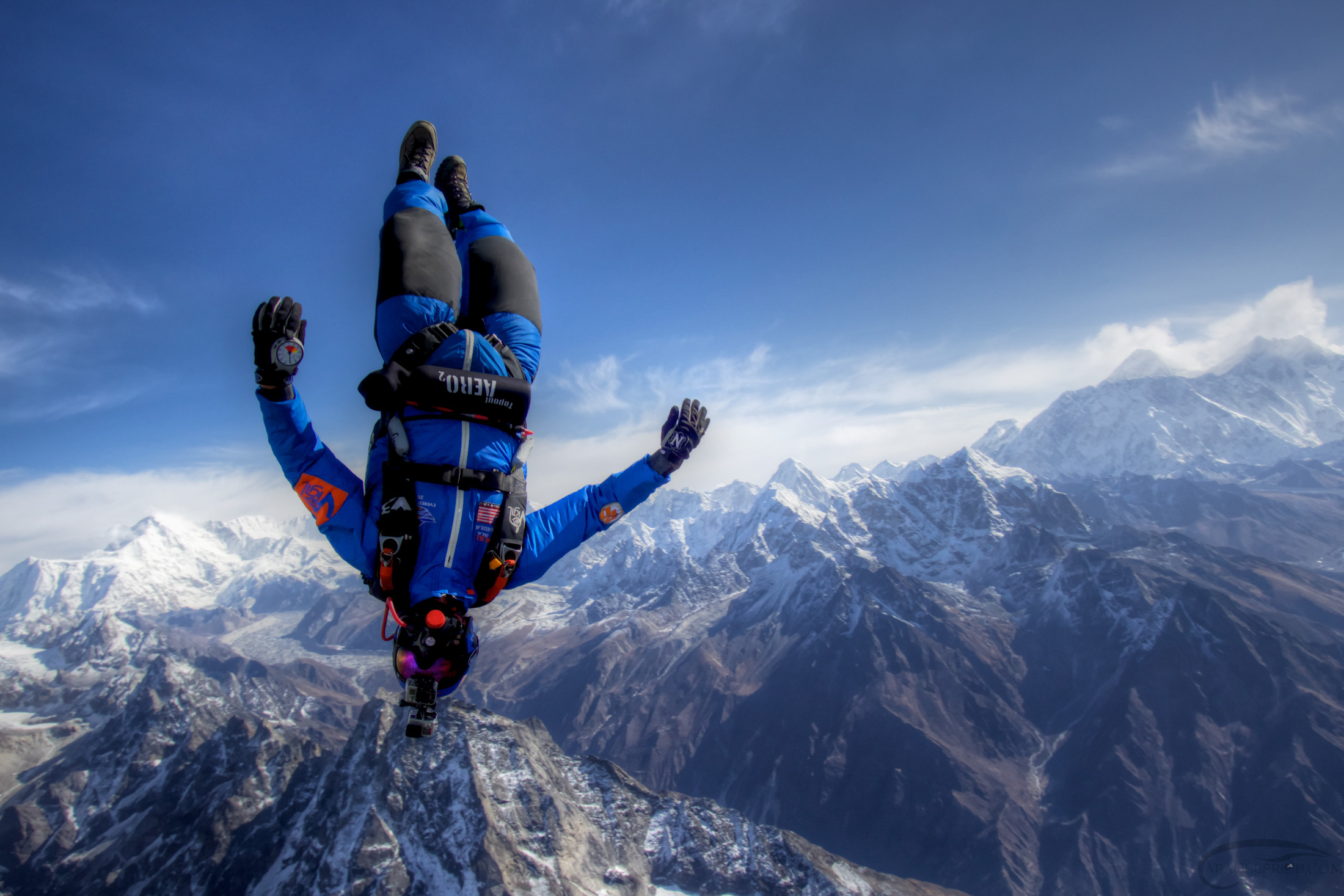In this breathtaking image, an upside-down skydiver clad in a connected blue puffy jumpsuit can be seen tumbling through a vibrant, medium-blue sky adorned with puffy white clouds. The skydiver is equipped with a grey GoPro action camera, notably strapped to their helmet, with a distinct black lens and handle. A prominent black skydiving backpack, marked "Arrow 2," is anchored around their waist, belly, and crotch. His outfit is further detailed with various brand patches and black padded areas over the knees, adding to the overall rugged look.

The skydiver's footwear consists of grey and brown boots, while his hands are outfitted with mismatched gloves: a thick black glove on his left hand and a skinny grey and purple glove on his right. Below, a vast mountain range stretches across the horizon with multiple peaks, some adorned with a picturesque layer of snow. The mountains exhibit a palette of blue and dark grey tones, contrasting against the sky. In the backdrop, an expansive valley nestles what appears to be a body of water, adding depth to the stunning scenery.